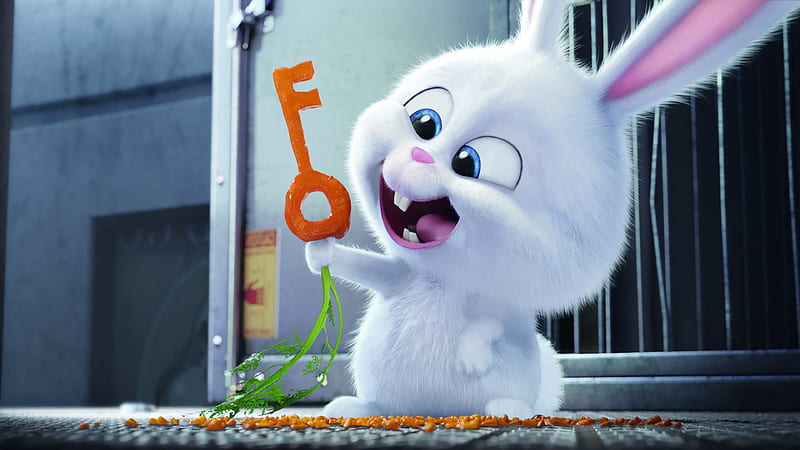The image is a color-rectangular still from an animated film, possibly from "The Secret Life of Pets," and it features a small, happy cartoon bunny centered in the frame. This adorable white fuzzy rabbit, with bright pink ears edged in mauve and big gazing eyes, is holding a carrot that has been creatively chewed into the shape of a key. The carrot, orange with a green stalk pointing downwards, is surrounded by chewed carrot bits scattered on the metallic ground at the bunny's feet. The background is a dark gray, industrial setting, suggestive of a cage or building with a warning sticker affixed to a metal surface, emphasizing the contrast with the vibrant, cheerful bunny and its innovative escape tool. The cropped ears at the top of the frame add to the whimsical feel of the image.